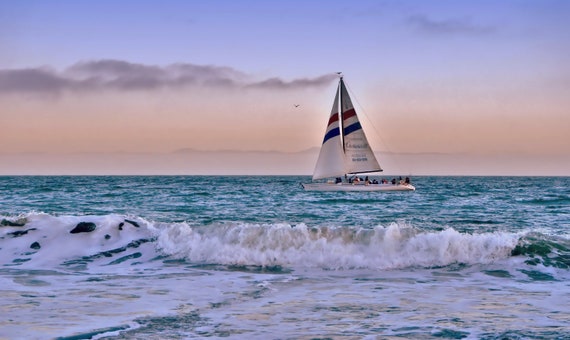This horizontal rectangular photograph captures a dynamic scene of a sailboat navigating choppy, light blue waters with waves cresting near the shore. The beach where the viewer stands features a prominent wave rolling in, accompanied by scattered rocks on the right side. The white sailboat, positioned centrally on the lake, has two distinct white sails, each adorned with a black stripe toward the top. While details about the occupants are unclear, there appears to be a number of people on board, suggesting active use. The lively water surface, marked by numerous white oxygen bubbles, indicates the presence of strong, energetic waves. The horizon line showcases a serene blend of light pink and purple hues with wispy gray clouds, transitioning upward into a deepening blue sky.